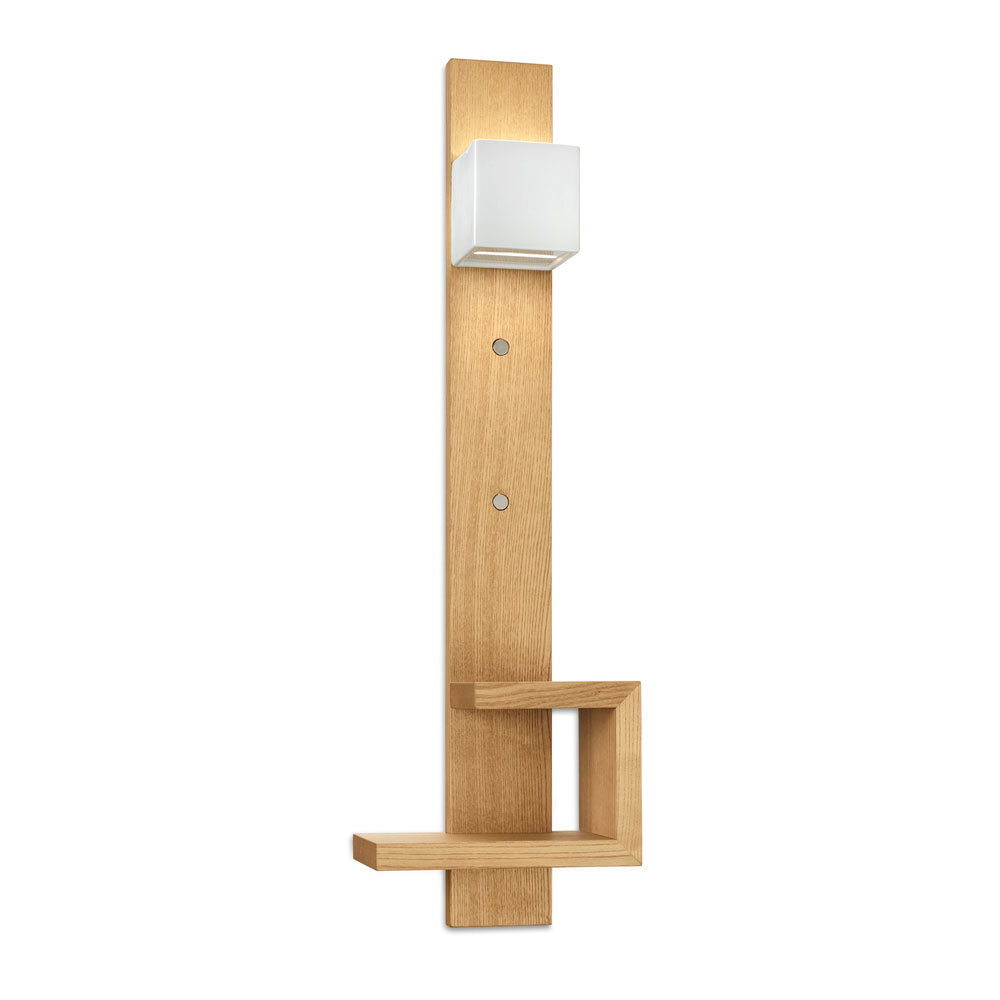The image features a vertical, light-colored wooden plank, clearly intended for wall mounting. At the top of the plank, there is a white plastic housing that appears to be a light fixture, emitting light from its top and bottom. Just below this light fixture are two small, round silver screws positioned one above the other, likely serving as mounting points. The bottom portion of the plank showcases a geometric, rectangular structure resembling a small shelving unit, with a longer horizontal board at the base and a shorter one above it, connected by a vertical piece, creating a cuboid form.